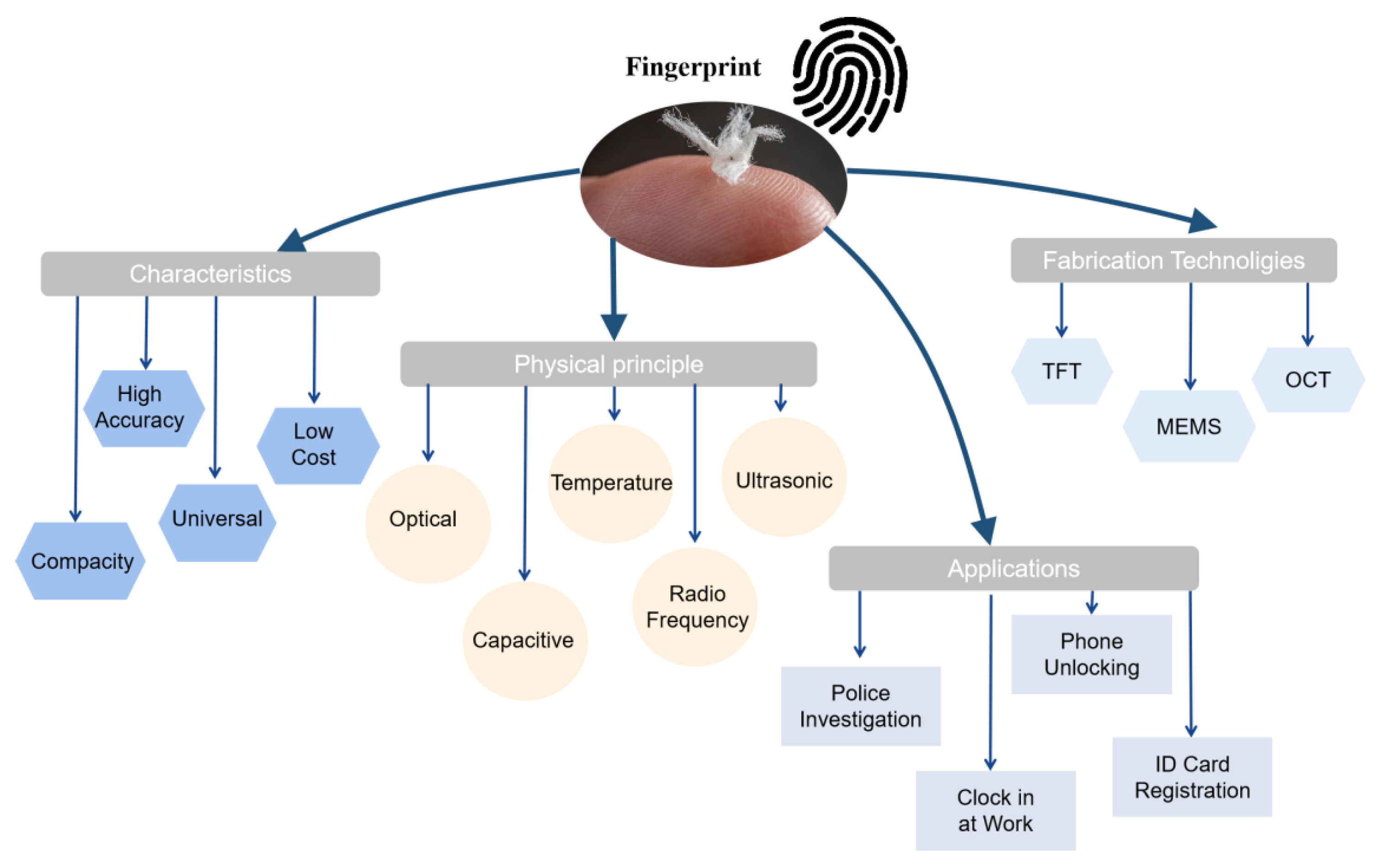The image is a detailed flowchart with a white background, prominently titled "Fingerprint" at the top, accompanied by a black fingerprint icon. Below this title is an oval graphic depicting what appears to be a fingerprint partially covered by a piece of white cloth or fuzz. This central fingerprint image has four primary arrows branching out.

The first arrow, leading to the bottom left, points to a gray box labeled "Characteristics." From here, further blue arrows extend to additional blue boxes listing specific traits: "compact sensitivity," "high accuracy," "universal," and "low cost," all written in black text.

The second arrow directs rightward to a gray box titled "Physical Principle." This box outlines various methods: "optical," "capacitive," "temperature," "ultrasonic," and "radio frequency," all marked within yellow circles containing black text.

A third arrow descends to a gray box captioned "Applications." Inside this box are terms denoting different uses: "police investigation," "clocking at work," "phone unlocking," and "ID card registration," each linked by further arrows.

The final arrow points to a gray box labeled "Fabrication Technologies." This section breaks down into light blue pentagons listing "TFT," "MEMS," and "OCT," again specified in black text.

Overall, the flowchart comprehensively breaks down the characteristics, physical principles, applications, and fabrication techniques related to fingerprint identification, distinctly mapped out with color-coded arrows and boxes.